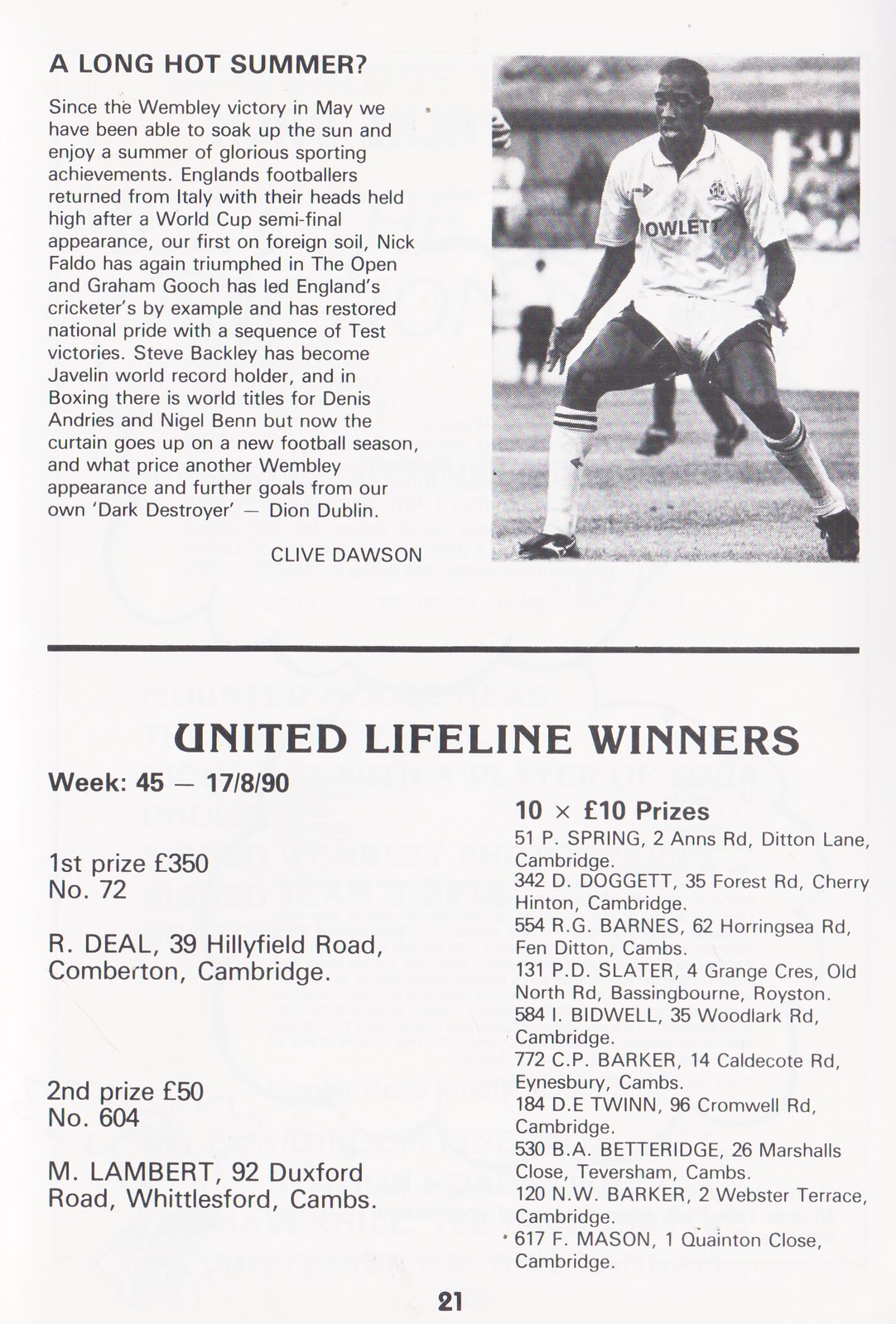A clipping from a magazine or newspaper features a monochromatic design with a light gray background. In the upper-right corner, a black and white photograph of a black man, likely a footballer, is positioned. He is slightly hunched over, wearing a white shirt, white shorts, white socks, and black shoes. This image accompanies a paragraph on the left, celebrating England's summer of sporting successes following the Wembley victory in May. It highlights England's footballers' semi-final appearance at the World Cup in Italy, triumphs by Nick Faldo in golf, and Graham Gooch's leadership in cricket. Additionally mentioned are Steve Backley's new javelin world record and world boxing titles won by Dennis Andries and Nigel Benn. The narrative then shifts to the anticipation of the new football season, questioning the prospects of another Wembley appearance and more goals from Dion Dublin, referred to as the 'Dark Destroyer.' This section concludes with the byline of Clive Davis.

Beneath this write-up, a bold black bar spans the width of the clipping, with text below detailing the "United Lifeline Winners." The left column lists the first prize of £350 awarded to entry number 70, located at Ideal, 39 Healyfield Road, Comberton, Cambridge. The second prize of £50 is awarded to entry number 604 at 92 Duxford Road, Whistleford Cabs. Additional smaller prizes of £10 each are also noted, with multiple entries such as 51 Pea String, 2 ANS, Roe Denton Lane, Cambridge, and concluding with 6-17-F Mason, 1 Quainton Close, Cambridge. The bottom right of the clipping displays the number 21, centered.